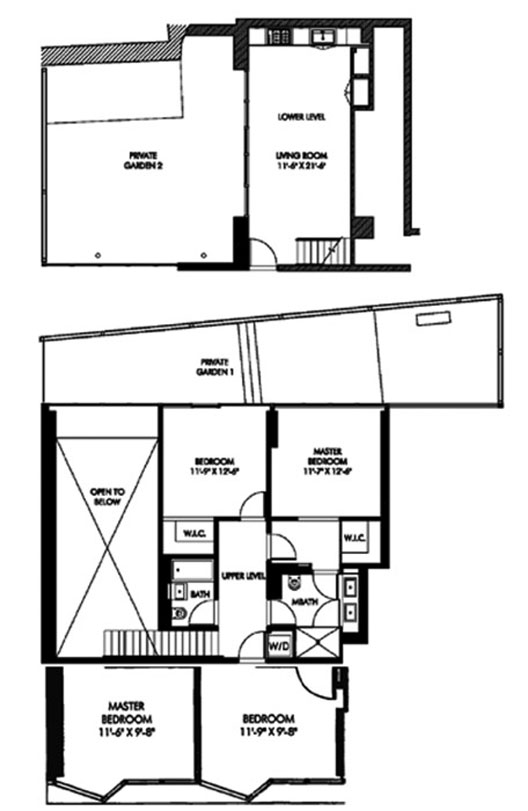This blueprint illustrates a building divided into two sections: the top portion represents the first floor, while the bottom portion corresponds to the second floor. On the first floor, from left to right, there is a sizable area designated as a "Private Garden," clearly labeled for both sections. Adjacent to the garden is a large rectangular space marked "Lower Level Living Room" with dimensions noted as approximately 11' X 21', although the text is somewhat small. 

The blueprint also highlights stairs that lead to the second floor. The second floor features spaces labeled "Private Garden," an area "Open to Below," and bedrooms including a "Master Bedroom" and an "Upper-Level Master Bedroom." Each area is precisely labeled with clear indications for spatial orientation and functionality.